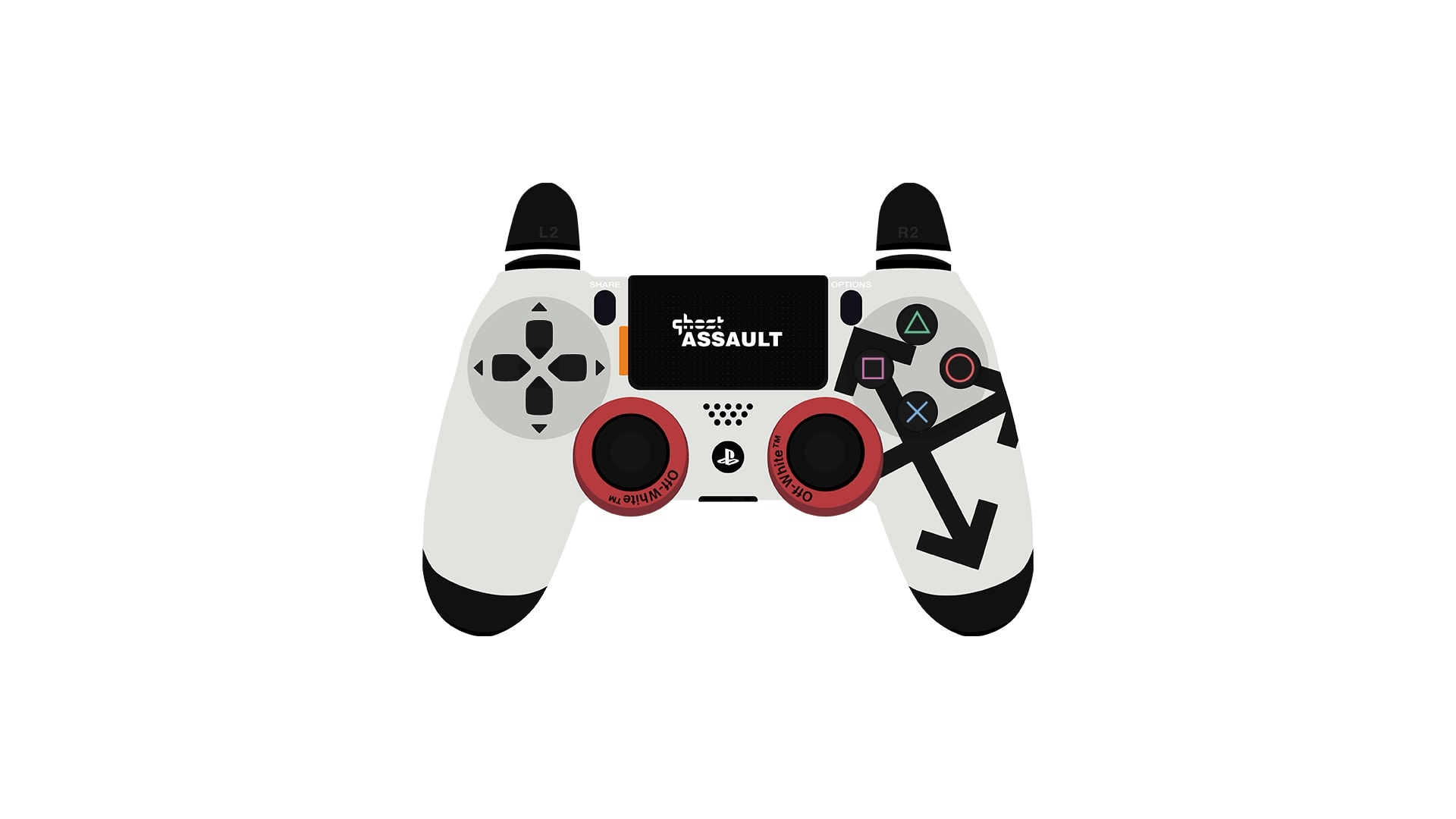This image showcases a product shot of a PlayStation controller, appearing to float on an all-white background. The controller, designed for two-handed use, prominently features a black and white color scheme with red accents. The body of the controller is predominantly white, with black covering the bottom and top tips, as well as the L2, L1, and R2 buttons. The controller's buttons are familiar to gamers: the triangle, square, circle, and cross symbols, colored in green, blue, red, and purple respectively, located on the right side.

In the center, the touchpad area displays the text "Ghost Assaults," indicating that this controller might be themed for a specific game. Below the touchpad are two red circular surrounds around the joysticks, which also bear the small and somewhat difficult-to-read text "off-white TM." The overall design includes a crossed arrow D-pad on the left side, completing its appearance as a specialized, functional PlayStation controller.